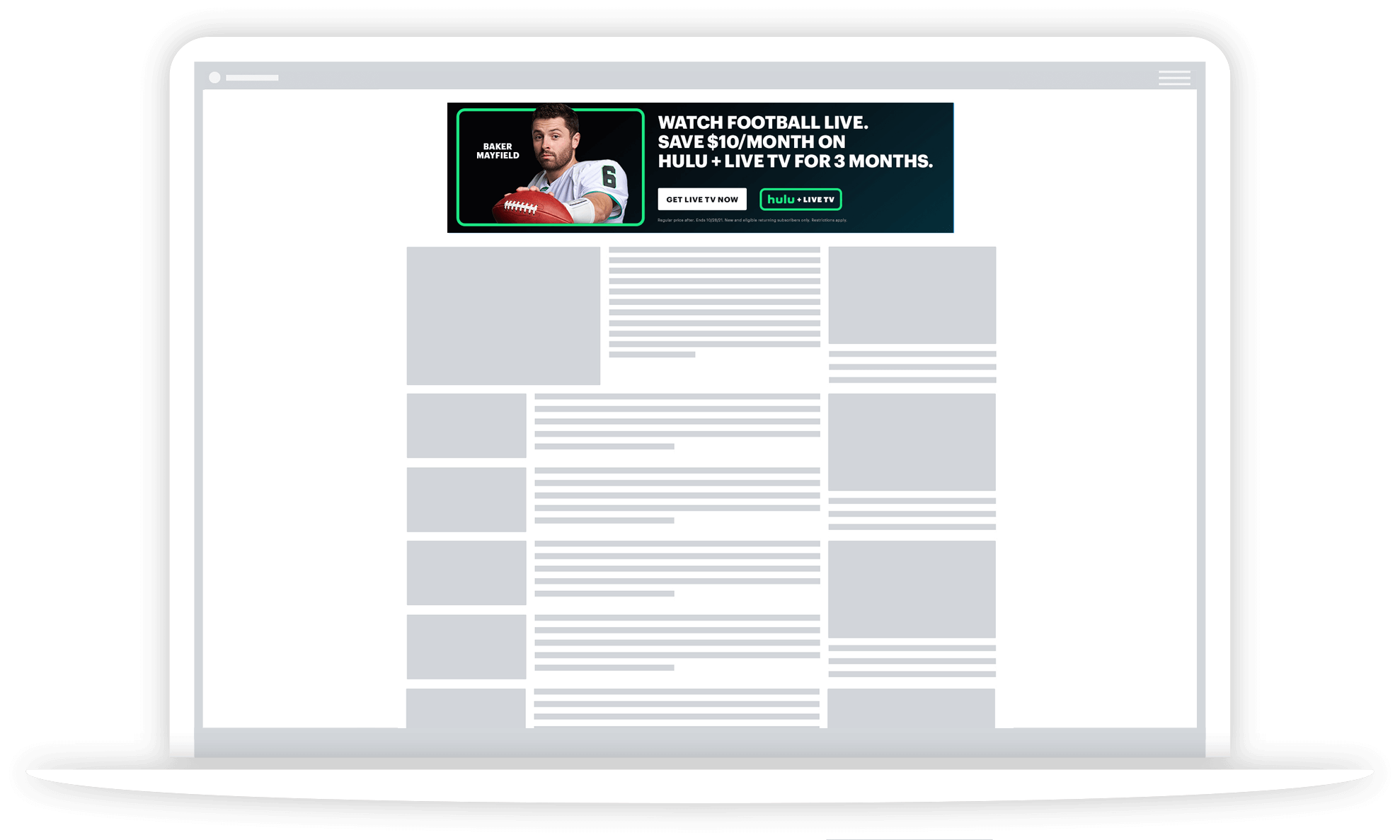The image appears to be a digitally rendered or hand-drawn representation of a laptop screen displaying a simplified web page layout. The screen background is grayed out with a light gray border. The main section is divided into various elements:

- **Left Column:** The left-most column contains a vertical arrangement of six gray rectangles, resembling placeholders for images or icons. The top rectangle is the largest, and the remaining five are slightly more than half its size in both length and width. The bottom rectangle is only partially visible, as if cut off.

- **Center Column:** The central section features several horizontal lines, mimicking text placeholders. These lines extend the full width of the column, suggesting areas where written content would normally appear.

- **Right Column:** The right-most section contains three and a half larger gray rectangles. These are smaller than the largest one in the left column but larger than the other five. Beneath each of these, there are three more horizontal lines, similar to those in the center column, likely indicating additional text placeholders.

- **Header:** At the very top of the screen, there is a blue rectangular bar that stands out as the only colored element in the image. It contains a green outlined rectangle within which is a head-to-chest image of a football player holding a football. The player's name is indistinct but might be 'Baker' or 'Mansfield'. 

  Next to the player's image, there's a promotional text in white: "Watch football live save $10 a month on Hulu plus live TV for three months." Below this, a white bar, whose text is unreadable, spans the width, accompanied by a green bar labeled "Hulu" towards its right end.

Overall, the layout implies a mock-up design used perhaps for wireframing a web page, with specific emphasis on hierarchical structure and spacing.